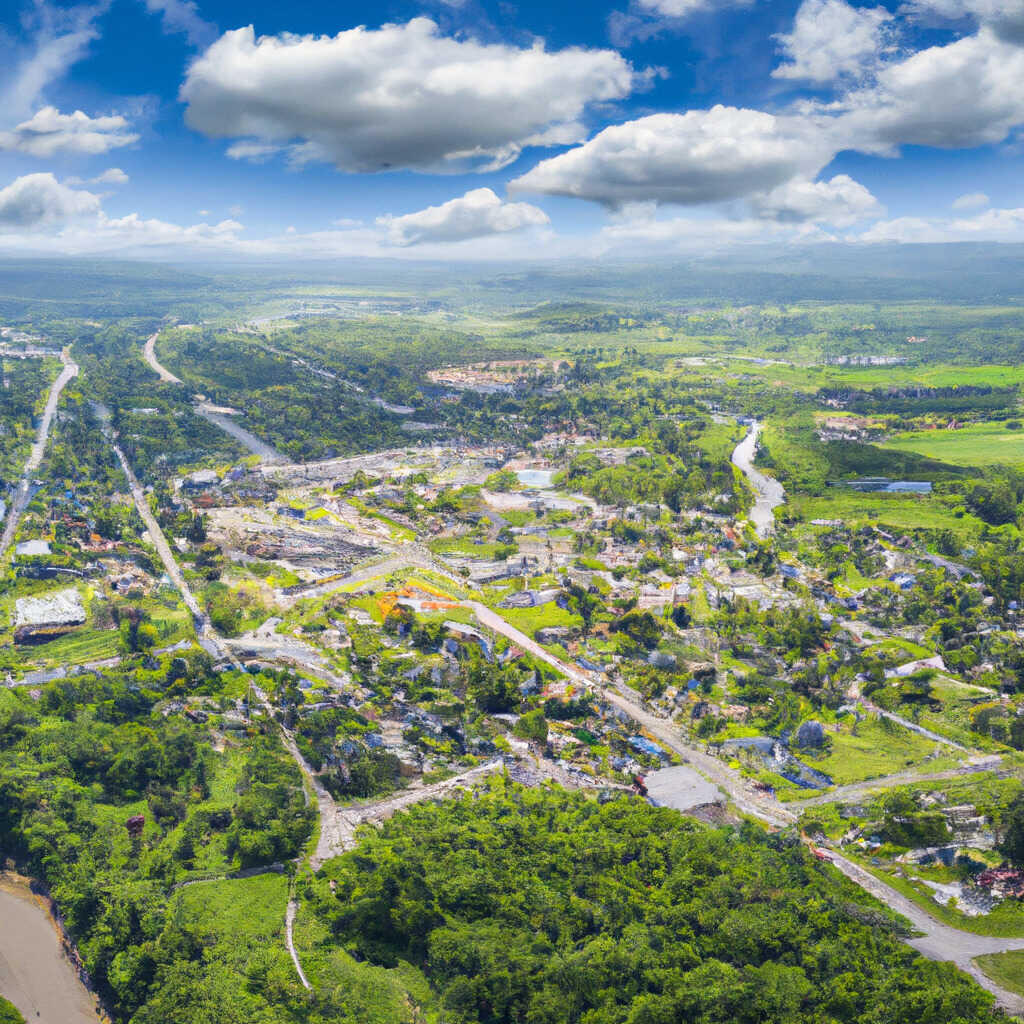This is an aerial photograph capturing a vibrant, extensive countryside from a high vantage point, looking down at an angle. The bright blue sky in the upper part of the image is interspersed with various types of clouds, including white and gray-bottomed storm clouds, stretching into the horizon until merging with a distant cloud line. The landscape below is rich with green hilly areas, abundant trees, and dense brush. Prominently, the image features a meandering river and possibly another parallel waterway cutting through the scene. Several roadways intersect the lush terrain, extending as far as the eye can see, winding through different types of houses and buildings scattered across the area. In the foreground, there's a large clearing with vibrant green spaces, grassy patches, and trees, forming a prominent spot where most buildings are concentrated. A mountain range is visible in the background, particularly on the right, adding to the picturesque quality of the scene, while patches of lime greens, yellows, and oranges dot the landscape, contributing to its vividness.